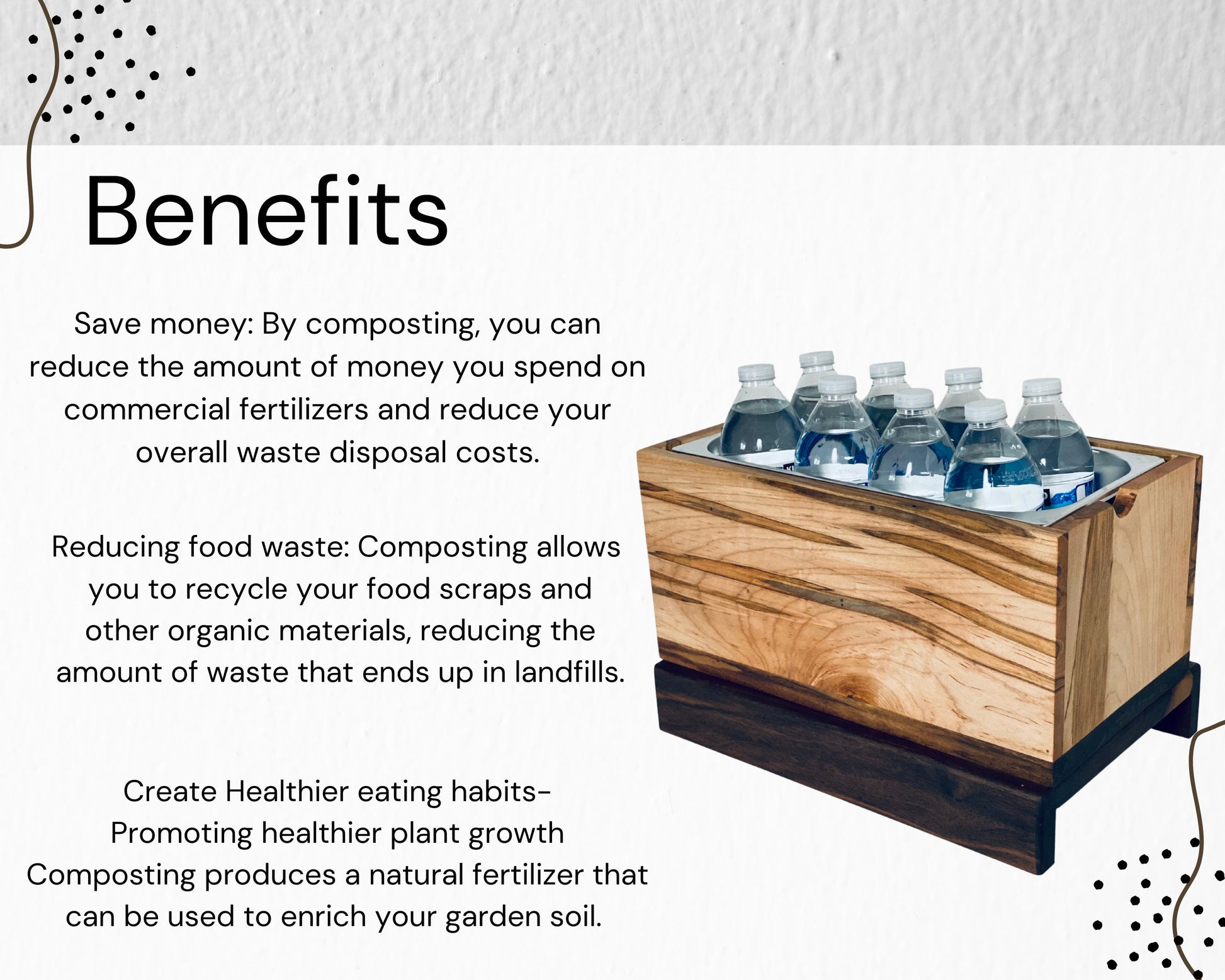The image is a detailed design highlighting the benefits of composting, featuring a clean, white background with a rectangular gray top section adorned with a swirly line design and a series of small black dots. The central text, displayed in black font on a white backdrop, lists three main benefits of composting: saving money, reducing food waste, and promoting healthier eating habits through healthier plant growth. These benefits are elaborated as follows: composting helps reduce expenses on commercial fertilizers and waste disposal, allows recycling of food scraps and organic materials to minimize landfill waste, and produces natural fertilizer to enrich garden soil.

On the right side of the image, there is a light wooden box with a dark wooden base and legs, containing eight visible water bottles, symbolizing the savings achievable through composting. Additionally, a small black design in the bottom right mirrors the one in the top left, creating a balanced visual aesthetic reminiscent of a PowerPoint slide layout.